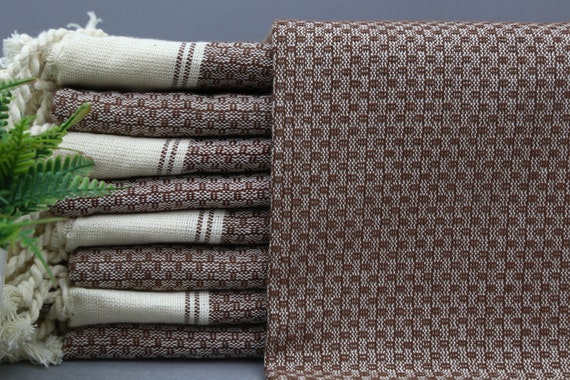The rectangular photo, oriented with the long sides on top and bottom, features a neat indoor arrangement against a light grayish-blue background. On the left side, fern leaves slightly intrude into the frame. The central focus of the image is a meticulously folded stack of fabrics that closely resemble either napkins or a blanket. These fabrics display a detailed brown and white pattern, characterized by alternating intricate dark and light brown rectangular weaves, tiny oval designs, and parallel dark brown lines on a white band along the edges. One prominent piece with rough white yarn ruffles on its edges is folded multiple times, with at least four visible folds, and a fifth piece draped over the top, showcasing the pattern clearly.